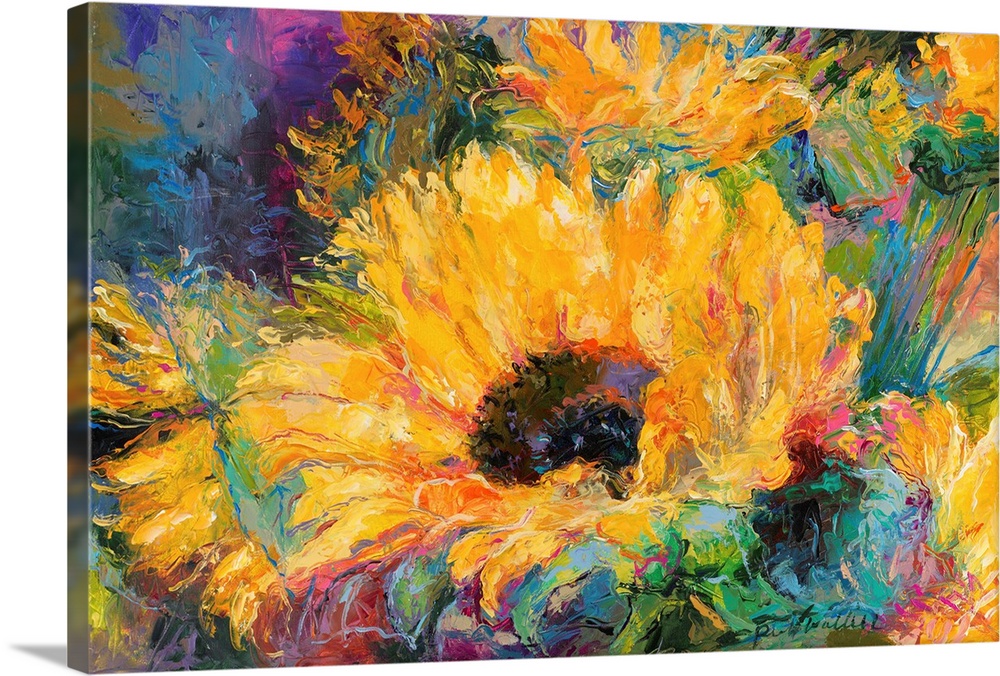This image features an oil or acrylic canvas painting of a vibrant floral motif. Dominating the center is a large flower with a striking black center surrounded by yellow-orange petals, exuding a sunflower-like vibe. This main flower captures the viewer's attention amid a background of smaller flowers and lively splashes of color. The composition includes a harmonious blend of greens, blues, purples, pinks, reds, oranges, and accents of black and white, creating a fresh and spring-like atmosphere. The artist's signature is delicately positioned in the bottom right-hand corner, though it is somewhat indiscernible. The painting's splotchy, abstract style uses bright and bold colors to achieve a captivating landscape.